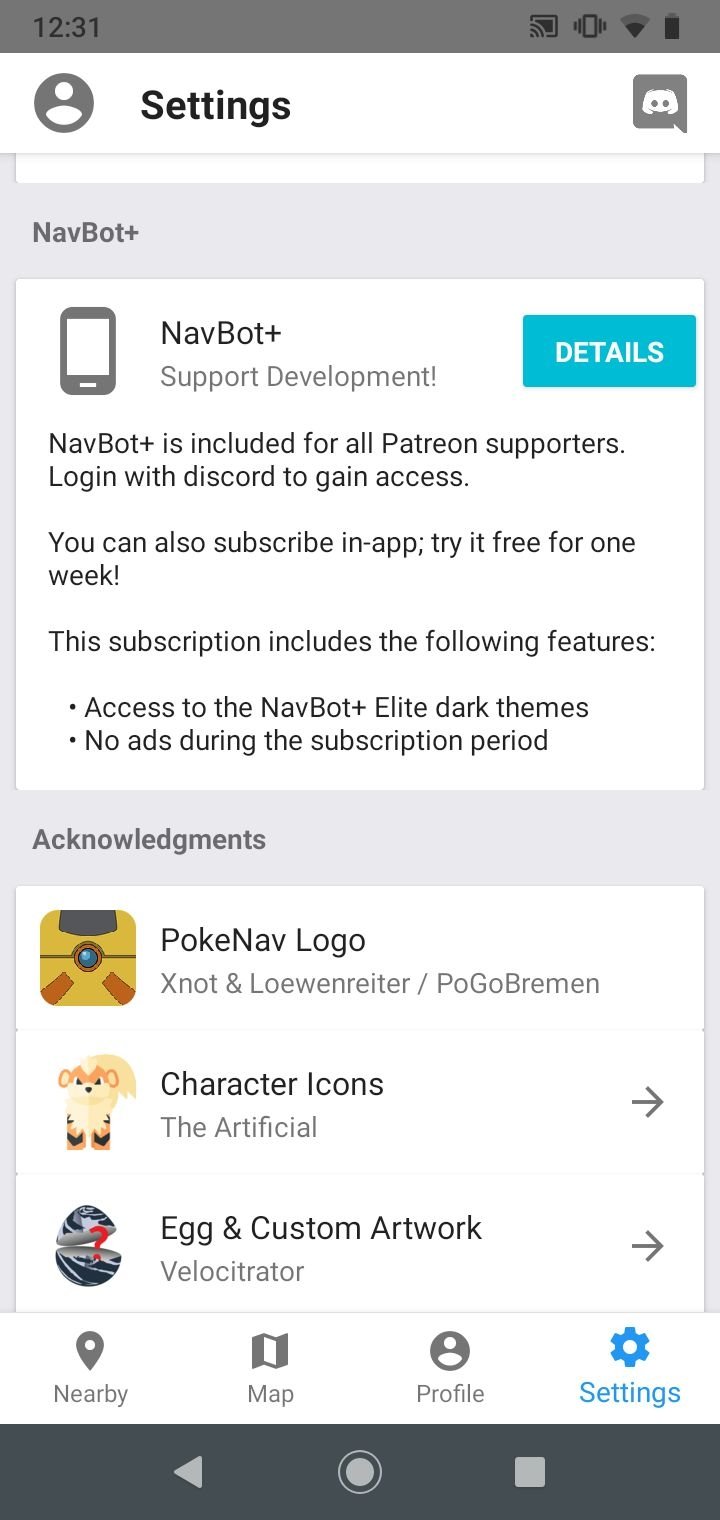Screenshot of an Android phone displaying the settings of a navigation app called NavBot. The interface is in light mode with a white background. There is a prominent section detailing an optional upgrade to "NavBot Plus," which is included for all Patreon supporters. Users also have the option to subscribe to NavBot Plus directly within the app, with a free trial available. Further down the settings, there is an "Acknowledgements" section mentioning the use of the PokeNav logo and character icons, which seem to suggest a custom artwork integration. This indicates potential collaboration or usage alongside the Pokemon Go app.